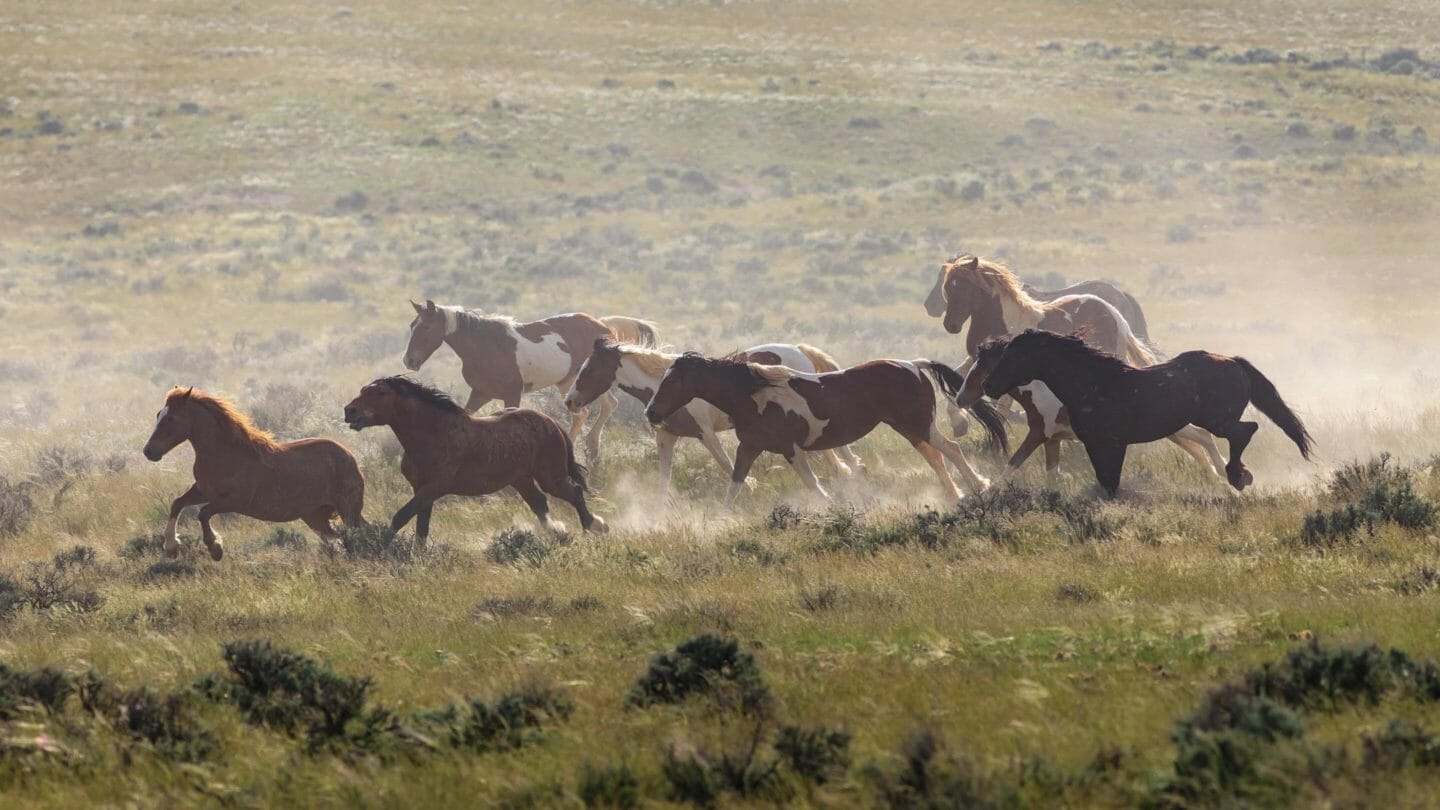In this stunning National Geographic-style photograph, a dynamic herd of wild horses, consisting of around ten majestic creatures, races across the grassy plains. Central to the image are the powerful strides of horses in varied hues, including solid brown, ebony black, and strikingly mottled with patches of brown and white. The horses, kicking up clouds of dust as they gallop to the left, create a sense of motion and energy. The landscape, lush with green grass and dotted with small shrubs, rolls gently with hills that give way to a more expansive, flat plain in the background. The scene is void of any man-made structures, emphasizing the untamed beauty of nature with the verdant valley stretching out beneath a partly clouded sky. The depth of field and the dusty mist add to the raw, unfiltered wildlife spectacle, making the herd the unmistakable centerpiece of this breathtaking moment captured in time.